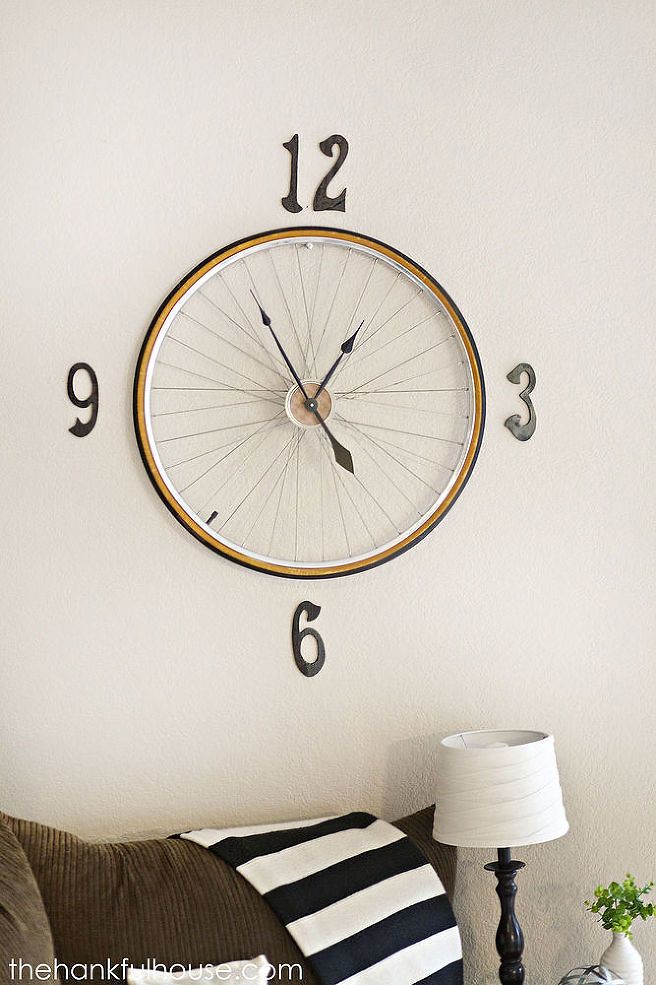This photograph captures a vibrant living room scene centered around a large, modern wall clock. The clock's minimalist design features only the numbers 12, 3, 6, and 9 affixed directly to the wall. Below these, a circular clock face displays the hour and minute hands, indicating the time as 4:50. Radiating from the clock's face are several light-colored spokes that add a dynamic, sunburst effect. In the foreground, a cozy couch draped with a striped blanket adds a touch of warmth and comfort to the setting. The overall composition of the room blends modern elegance with inviting homeliness.